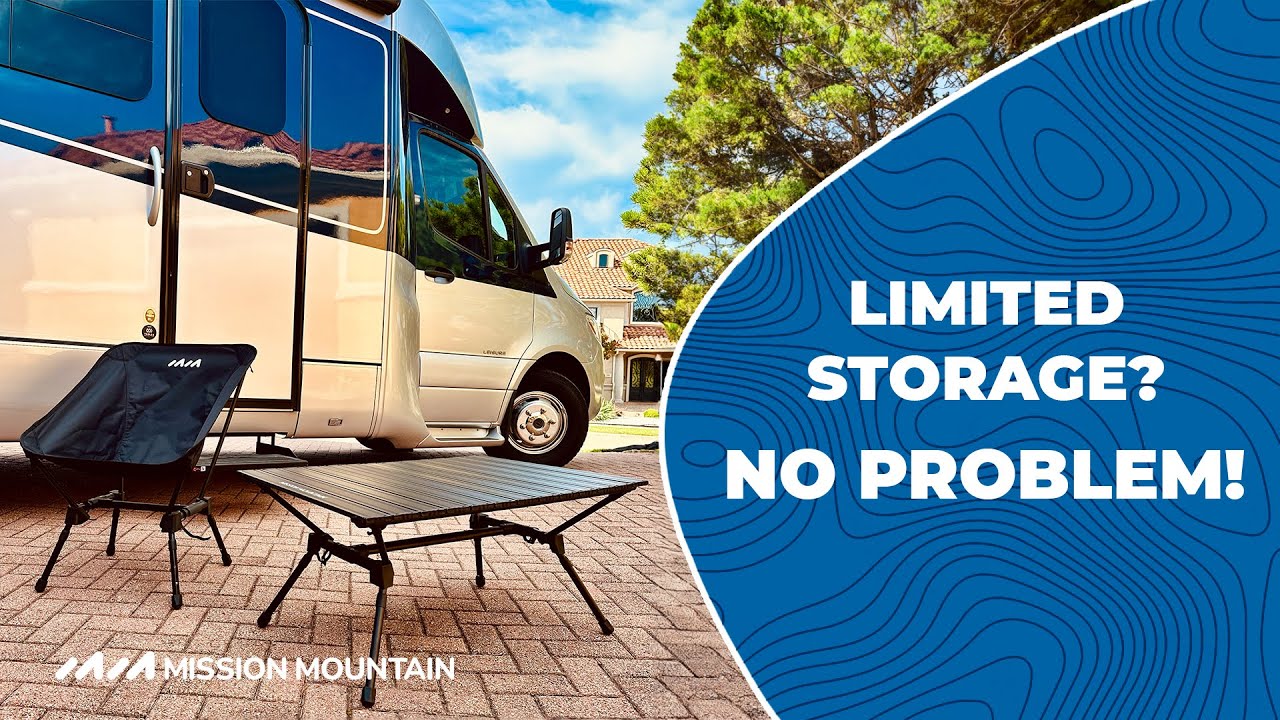The advertisement features a detailed photograph of a camper van, highlighting its beige and black design with white trim. Only the front right side of the van is visible, showcasing its silver wheels with black tires and both the passenger door and rear compartment door, each fitted with handles. In the foreground, a black camp chair adorned with unreadable white text and a small black square table are neatly arranged on a paver brick driveway. A Mediterranean-style house with a stucco roof and lush green tree foliage provide a scenic backdrop against a bright blue sky adorned with white clouds. On the right side of the image, a blue section with black swirly lines frames the bold white caption: "Limited Storage? No Problem!" The Mission Mountain logo and text are distinctly placed in the lower left corner of the photograph.